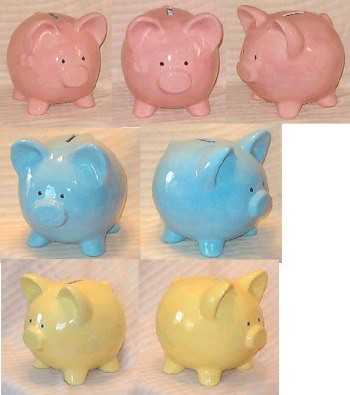The image showcases a collection of seven identical, round piggy banks arranged in three rows. Each piggy bank has a circular body, with two round, slightly pointy ears, a short stubby nose, and small black eyes. All piggy banks have four short legs and a slit on top for inserting money. The bottom row features two pale yellow piggy banks; the left one slightly oriented left and the right one angled towards the right. The middle row displays two piggy banks of the same design but in a light blue color, with the left one facing left and slightly towards the viewer, and the right one facing right. At the top row, there are three pink piggy banks, each depicted from different angles; one faces right, another slightly towards the viewer, and the third one left. This neatly organized grid of piggy bank images illustrates the same design in varying colors and orientations.